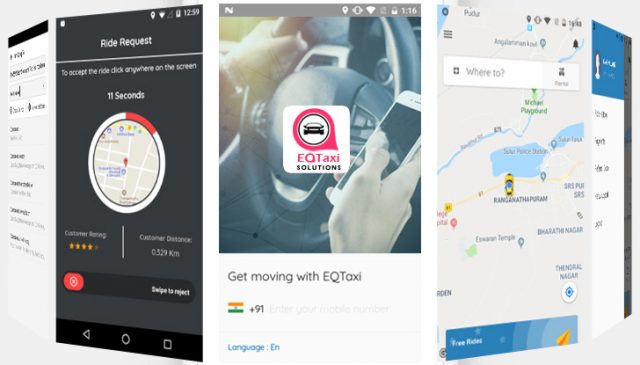The image is a collage of multiple screenshots taken from a mobile phone. 

- The first screenshot on the left displays an interface with a black banner on top. Below the banner, there is a white background divided into multiple sections, though the text within these sections is not legible.

- The second screenshot to its right features a black background with a central map icon highlighting a location. Part of the circle surrounding the location marker is colored red, and the text "11 seconds" is displayed above it. Below the map area is a rectangular button with rounded edges, featuring the text "EQ Taxi Solutions". At the bottom, the words "Get Moving with EQ Taxi" are visible, accompanied by an icon that resembles a flag and a "+91" area code for phone numbers, with "EN" indicating the English language option. The font for this text is blue.

- The third screenshot appears to depict an active GPS navigation map. The "Where to?" section is visible, and a yellow car icon is centered on the map, indicating a location.

- The final screenshot on the right includes an empty profile picture area, a blue banner at the top, a white section below, and some unreadable text.

Each image captures different features and interface elements of what appears to be a mobile application, likely related to a taxi or ride-sharing service.